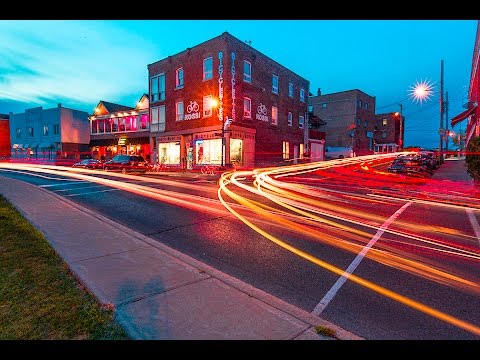The photograph captures a bustling street corner in a small town at dusk, just after the sun has set. The dark blue sky is becoming more vivid as the streetlights flicker on, painting a serene yet lively evening scene. Prominently featured is a three-story brick building adorned with the sign "Rossi" and a bicycle icon. This building, aglow with neon reds and oranges, stands next to a two-story structure boasting a large illuminated patio. Both buildings' interiors are lit, though their exact contents remain obscured.

To the left of the photo is a sidewalk bordered by a small grassy area, gently illuminated by the streetlights. The street itself is a symphony of motion, with light trails from passing vehicles creating dynamic streams of yellow and pink that curve around the corner, suggesting a vibrant flow of traffic. A mysterious starburst effect, possibly from a nearby streetlight or distant fireworks, adds an additional touch of enchantment to the scene. Parked cars are visible, grounding the composition in everyday life, while the overall effect is enhanced by skillful photo editing, which blurs the moving lights but keeps the rest of the scene in sharp focus.